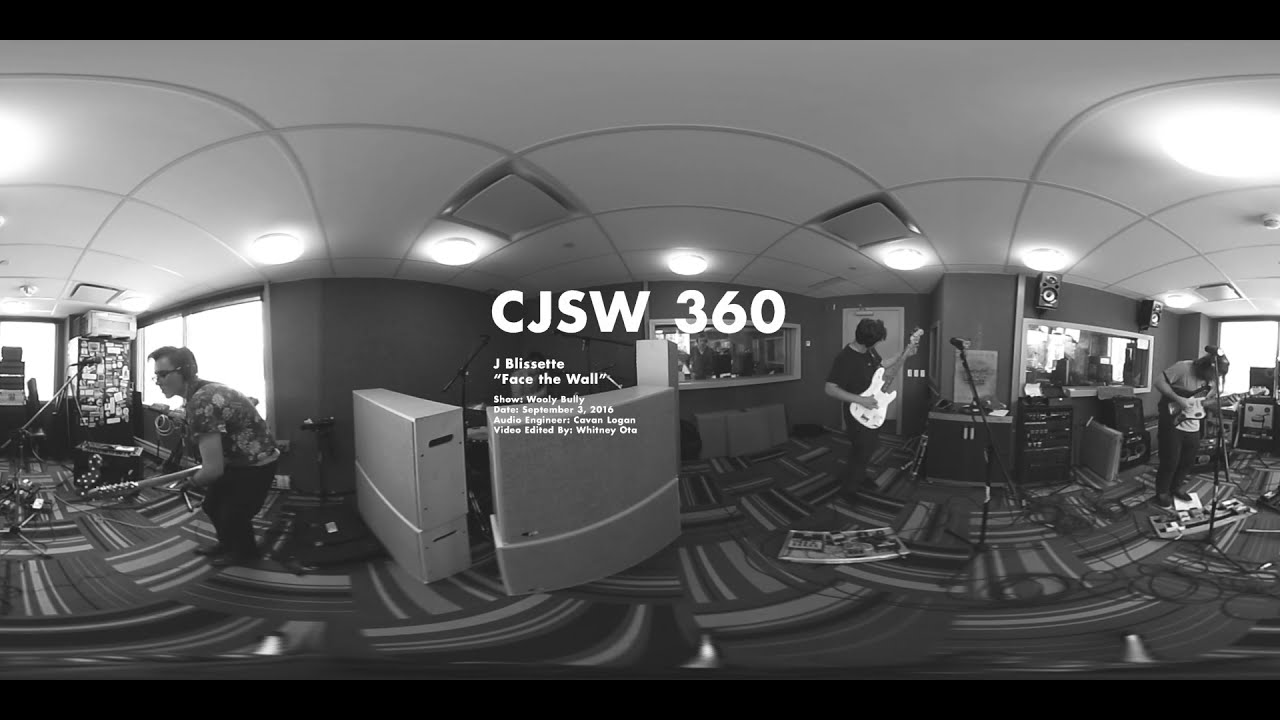The black-and-white image features several men inside a large recording studio, each playing a guitar. The rectangular, horizontal photograph has thin black stripes running across the top and bottom edges, framing the scene. Prominent white text overlays the center of the image, reading "CJ SW 360." Directly beneath this in smaller font, it reads "Jay Blissett," followed by the phrase "Face the Wall." Four additional lines of text detail the information about the date, personnel, and other production credits, although these are difficult to discern. Positioned under the bright studio lights, the man in the center wears a black short-sleeved shirt and plays a white guitar. On the far right, another man plays a guitar with a distinct border, donning a lighter-colored shirt. The man on the far left, partially obscured by his instrument, wears a shirt with intricate designs and glasses. The setup includes microphones and a multicolored rug on the floor, enhancing the studio ambiance, while observers watch from behind a glass window.